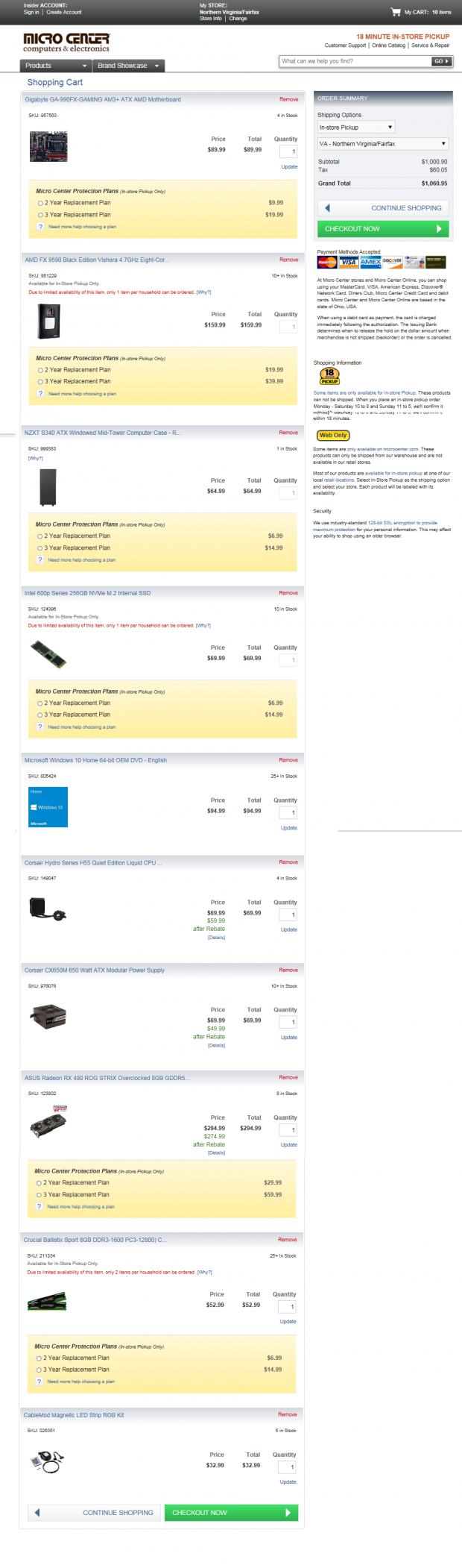This low-resolution vertical portrait-style image features a web form from Micro Center, a retailer specializing in computer hardware and electronics. Despite the clarity being highly compromised, certain elements can still be discerned. At the top, a black banner displays text that is indistinguishable due to the poor image quality. Below this banner, the recognizable Micro Center logo is displayed, accompanied by a tagline that is illegible.

Under the logo, the image showcases various product listings, though the specifics such as prices and product names are unreadable. Adjacent to these listings, on the right side of the image, is an ordering information section where users can input their shipping details and proceed with the checkout process.

The shopping cart section appears to contain several PC components, including what looks like a motherboard, RAM modules, a video card, storage devices, and possibly some cables. However, due to the low resolution, identifying each item with precision is challenging. Overall, this image reflects an online shopping interface from Micro Center, illustrating the steps involved in arranging the purchase and shipment of computer parts and accessories.